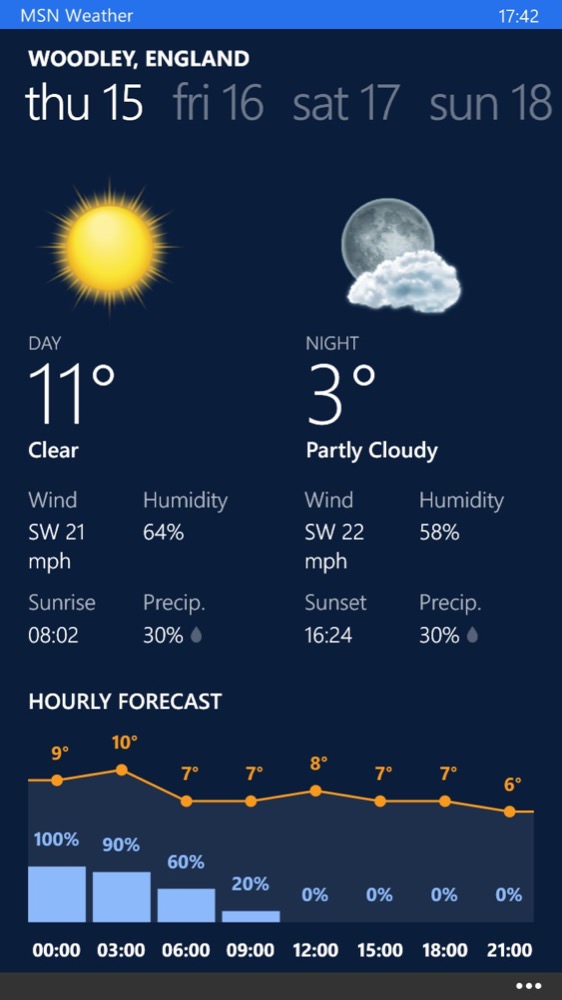This image showcases the mobile app version of the MSN Weather app, specifically displaying the weather forecast for Woodley, England. The app's interface features a navy blue background, providing a clean and visually appealing contrast to the weather information presented. 

At the top, the app lists the days of the week from Thursday (abbreviated as "CCTHU") through Sunday, each accompanied by the corresponding dates. Below this section, there is an icon of the sun, which indicates the daytime weather conditions. Directly beneath the sun icon, the app displays the daytime temperature details for the specified days.

To the left of the sun icon's section, there is an icon of the moon partially obscured by a cloud, which signifies the nighttime weather conditions. The temperatures expected at night are shown underneath this moon and cloud icon.

Further down, the app introduces an "Hourly Forecast" feature. This section includes an orange line graph, marked with discrete dots at various points, denoting the temperature changes throughout the day. Beneath the graph, small squares likely represent additional details or hourly intervals.

Overall, the detailed layout of the MSN Weather app provides a comprehensive and easily navigable weather forecast for users in Woodley, England.